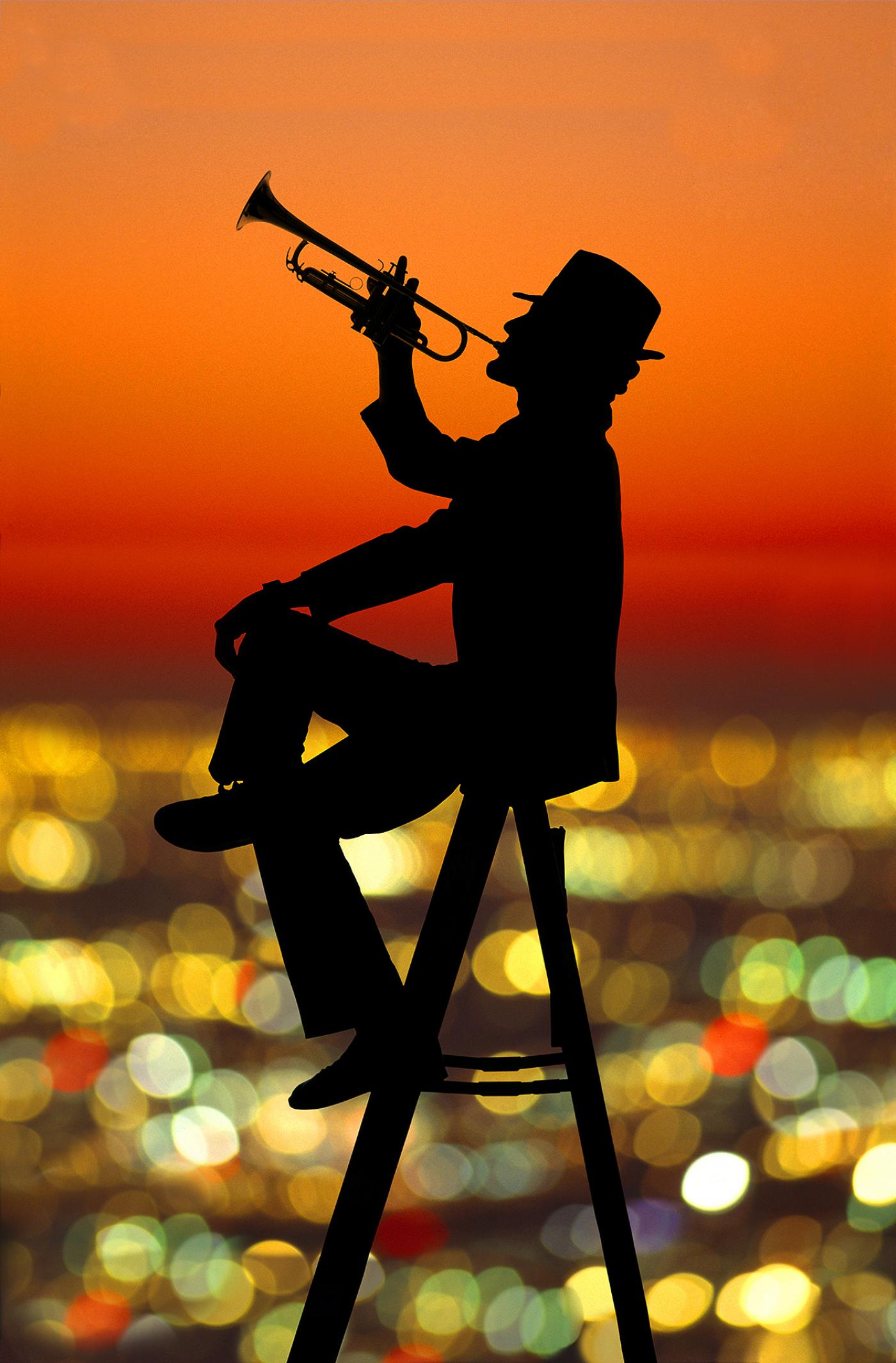The photograph captures a striking silhouette of a trumpet player at sunset. The sky above him is a mesmerizing gradient of glowing orange and red, while the lower portion of the image features a bokeh of out-of-focus, multicolored city lights, creating an ethereal backdrop. The central figure, entirely in black silhouette, is seated on what seems to be a tall wooden stepladder. He is wearing a rimmed hat and has his right leg crossed over his left, with his left foot resting on a rung of the ladder. His left arm is casually resting on his crossed leg, while his right arm is raised, bringing a trumpet to his lips. The silhouette is beautifully detailed, down to the slight contours of the hat and the poised posture of the musician, giving the impression that he is playing a joyful, heavenly tune into the glowing sky. The composition, combining the serene sunset with the vibrant out-of-focus lights, hints at a composite image, artfully blending these elements to emphasize the tranquil yet spirited moment.